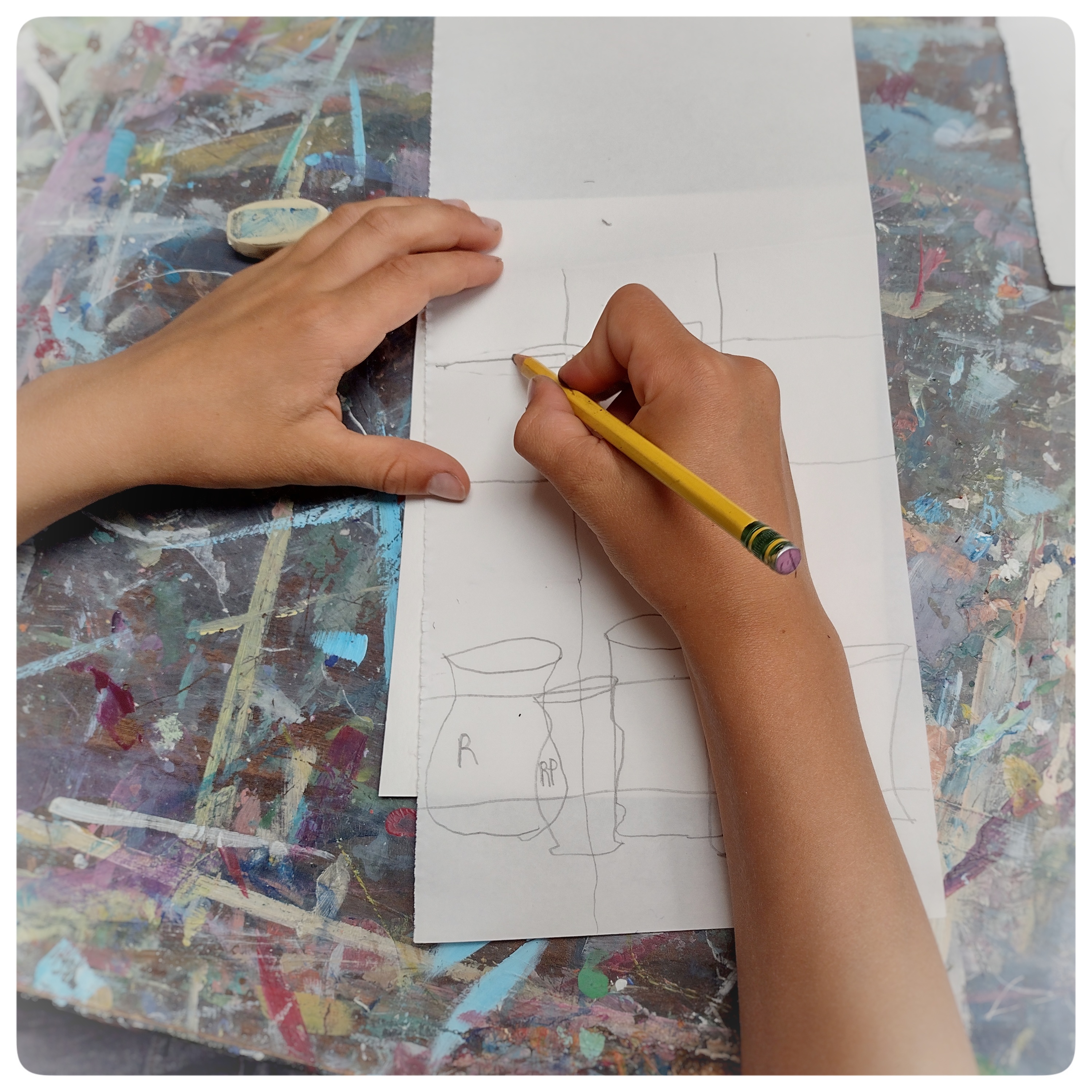A photograph captures a moment of focused creativity as a person, presumably a child, is engaged in drawing. The individual’s right hand, clutching a yellow pencil with black stripes and an eraser at its end, hovers over a partially completed sketch. Their left hand and forearm rest beside an orange eraser placed on a heavily marked workbench. The table surface is predominantly dark gray, but it is splattered with an array of colors, including whites, reds, turquoise, blues, and greens, hinting at numerous past artistic projects.

The drawing appears in a sketchbook, open in a portrait orientation, with a visible fold line near the person's left hand. The sketch itself consists of a grid layout featuring three columns of squares across and five rows down. Below this meticulous grid, the budding artist has begun to draw various shapes resembling vases, glasses, or pots. This detailed portrayal captures the essence of a creative workspace and the innocent concentration of youth immersed in art.